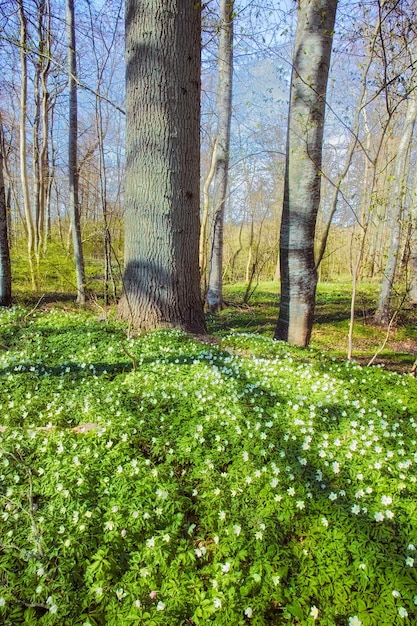The image captures a vibrant and serene outdoor forest scene, dominated by a dense array of tall and thin trees with varying bark colors ranging from light brown to gray, possibly due to the play of light. Some trees flaunt yellow-green leaves while others stand bare. The ground is a lush field of green grass dotted with numerous white flowers, each flower showcasing delicate white petals with a yellow center. Among the natural elements, a subtle walking path weaves through the forest floor enriched with dirt and occasional foliage. The background reveals glimpses of a blue, slightly cloudy sky, adding depth to the tranquil daytime setting.